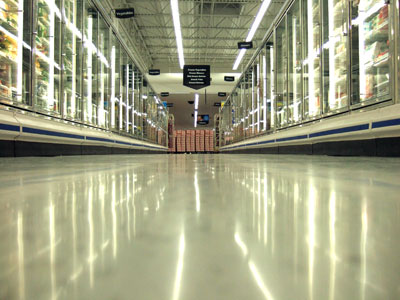The photograph captures a long freezer aisle in a large grocery store, possibly resembling a supermarket like Walmart. The picture is taken from a low angle, just a couple of feet off the highly polished gray-colored floor, which reflects the bright overhead lights. The aisle is flanked by rows of commercial-grade freezers on both sides, their glass doors revealing shelves filled with a variety of frozen products, though the exact items aren't discernible from the distance. The freezers have a distinctive design with white shelves and a base section embellished with black stripes and a black kick plate. Black placards hang at intervals above the freezers, indicating the types of products in each section. The high flat ceiling, covered with corrugated steel and exposed ceiling supports, adds to the industrial atmosphere of the aisle. At the far end of the aisle, there appears to be a stack of boxes or a pallet with packaging in a pinkish-red color, which could be food items or soda boxes. A large aisle sign with white text hangs from the ceiling, providing further navigation within this extensive grocery store.